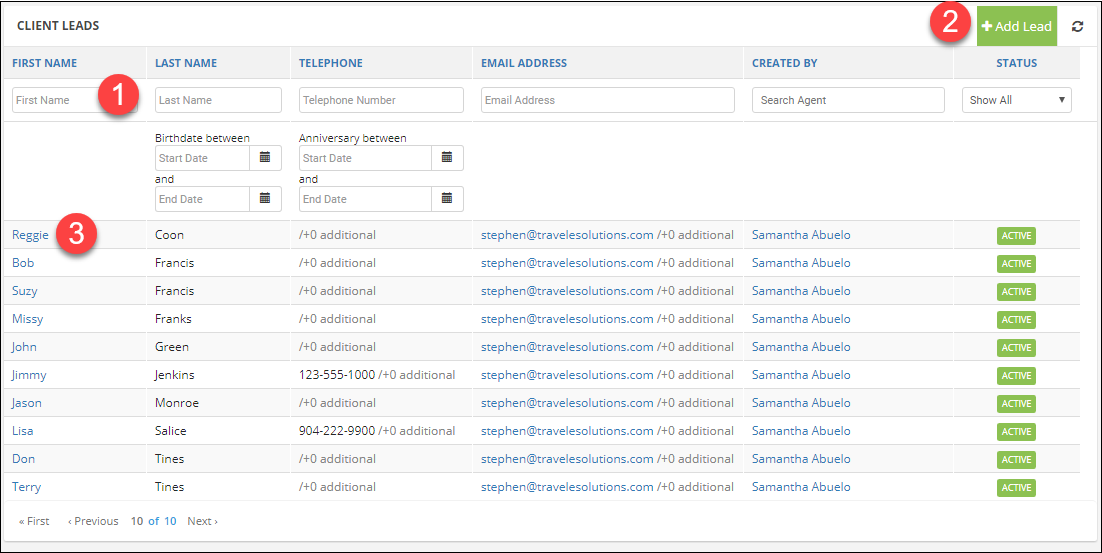The image displays a screen featuring a spreadsheet-style layout predominantly filled with text, and at the top, the header reads "Client Leads." Below this header, the spreadsheet is organized into several categories, which include First Name, Last Name, Telephone, Email Address, Created By, and Status. Directly beneath these categories, there are text fields available for entering information such as first name, last name, telephone number, and email address. The "Created By" field displays the search agent's name, and there's a dropdown menu to select the current status.

Additionally, the screen provides options to filter entries by birth date, anniversary dates, and both start and end dates. 

Displayed from top to bottom, the actual client leads listed are:
1. Reggie Kuhn
2. Bob Francis
3. Susie Francis
4. Missy Franks
5. John Green
6. Jimmy Jenkins
7. Jason Monroe
8. Lisa Salis
9. Don Tynes
10. Terry Tynes

Each of these leads shares the same email address: stephen@travelsolutions.com. Notably, the "Created By" field for all entries is attributed to Samantha Abuelo, and their current status is uniformly marked as "Active," indicated by a green button with the word "Active" in white text.